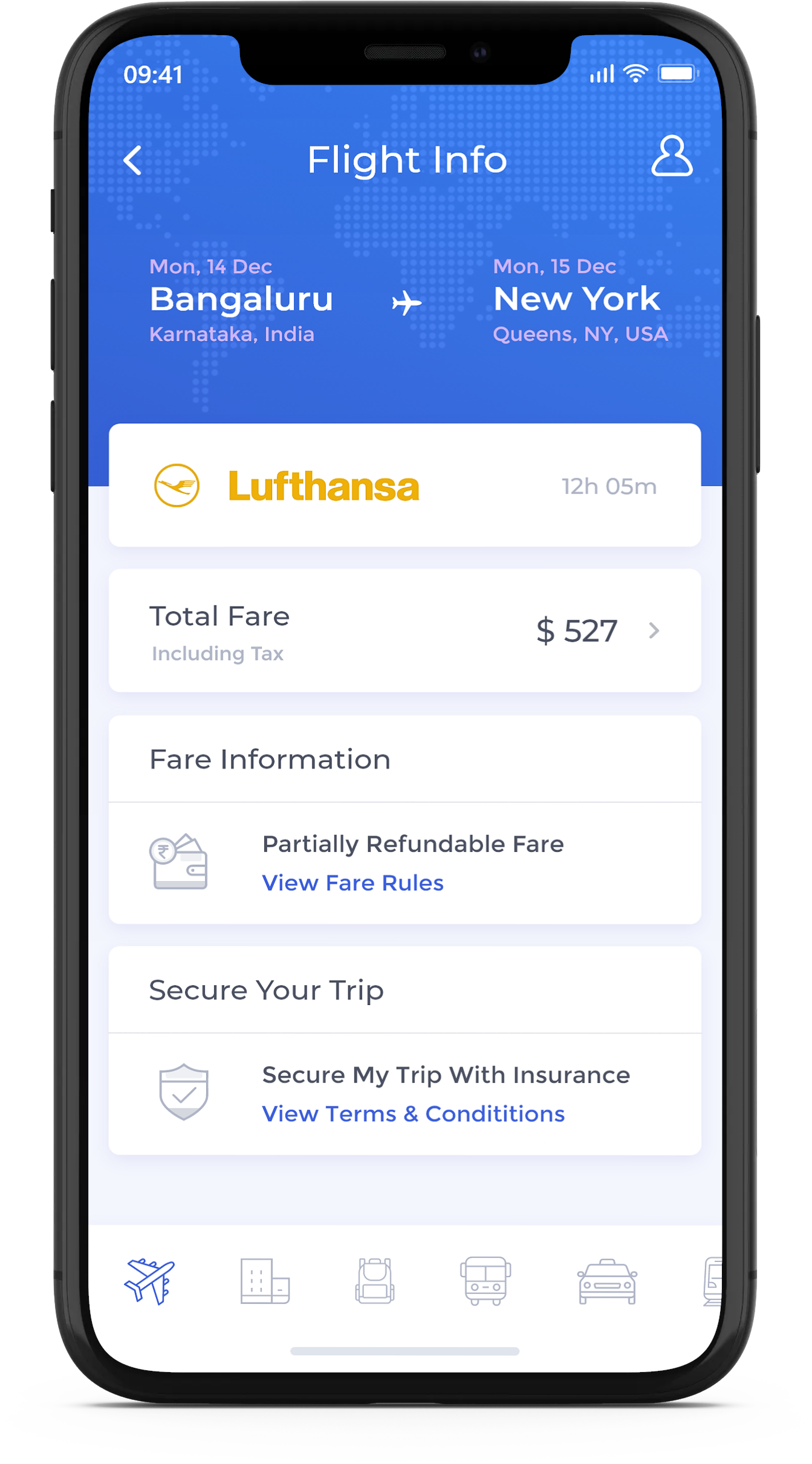This is a detailed screenshot of a cell phone displaying upcoming flight information for an individual. The phone appears to be a standard Android smartphone, characterized by three buttons on the left likely for power and volume control, and a larger button on the right. The screen prominently features flight details.

At the top of the screen, there is a blue background with a world map faintly visible behind it. The top left corner displays the time, 09:41. To the right, standard cell phone status indicators show signal strength, Wi-Fi connection, and battery life.

The main portion of the screen showcases detailed flight information, set against a backdrop that allows for navigation back to a previous screen and account management options. The flight is from Bengaluru (Bangalore), Karnataka, India to New York, Queens, USA on Monday, December 14th, arriving on December 15th. 

This flight is operated by Lufthansa and has a duration of 12 hours and 5 minutes. The total fare for this flight is $527, including taxes. Fare details indicate that the ticket is partially refundable, with clickable options to view fare rules, secure the trip with insurance, and review terms and conditions.

At the bottom of the screen, various travel options are presented, including icons for airplane, car, train, taxi, and an ambiguous building icon. The airplane option is currently highlighted.